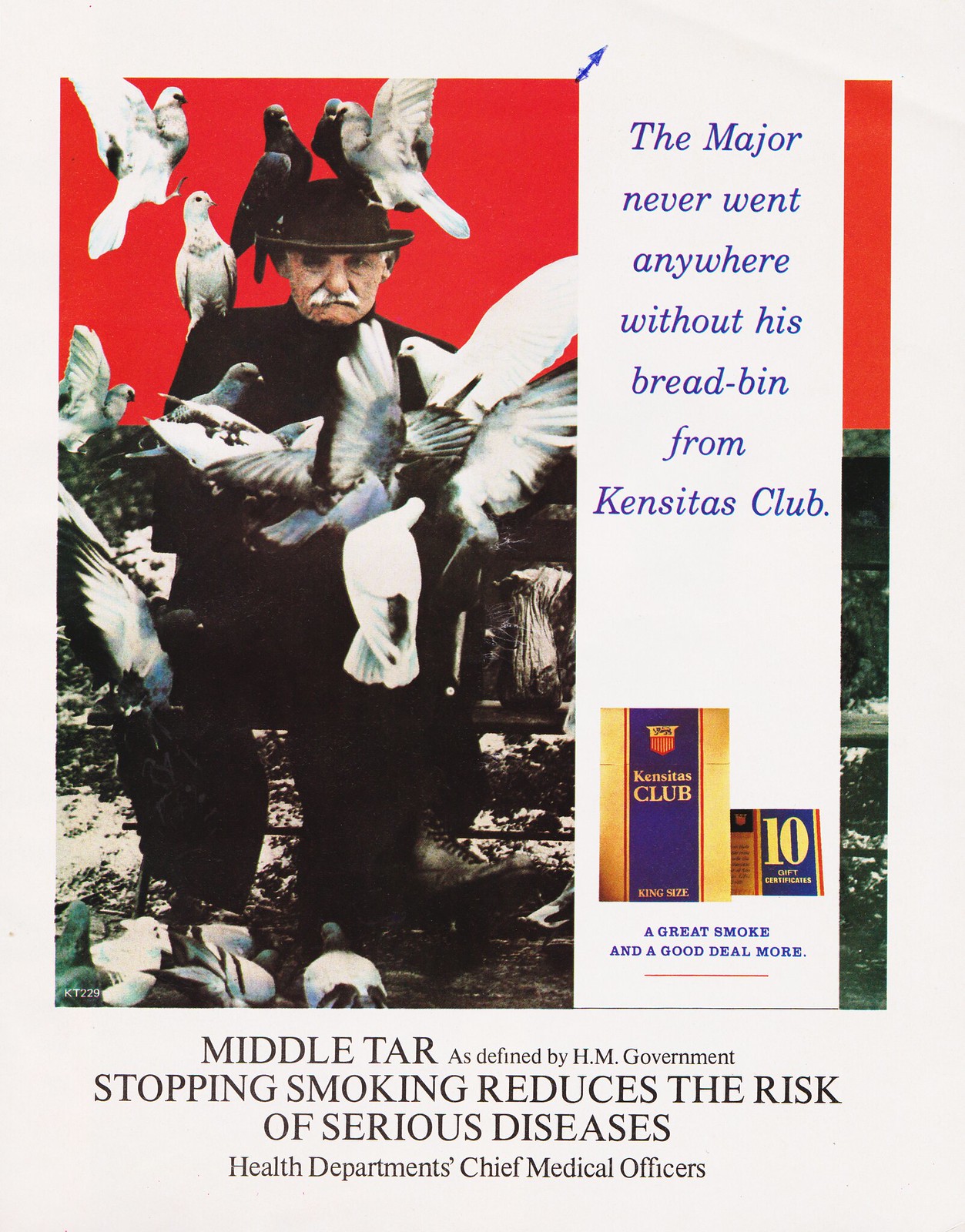The image is a vintage-inspired advertisement featuring an older Caucasian man with a white mustache, wearing a black top hat, seated on what appears to be a park bench. He is surrounded by numerous birds—four on his head, one on his shoulder, others perched on his lap, feet, chest, and several more in the process of landing. The man is facing forward with a displeased expression. 

The background is segmented, with the upper portion being a solid red and the lower part depicting an outdoor park-like setting. To the right of the image, there is text in white and blue that reads, "The major never went anywhere without his bread bin from Cancitas Club." Below this text is an image of a gold and purple cigarette package with blue accents, accompanied by the phrases, "a great smoke and good deal more," and "middle tar as defined by HM government. Stopping smoking reduces the risk of serious diseases," attributed to the Health Department chief medical officers.